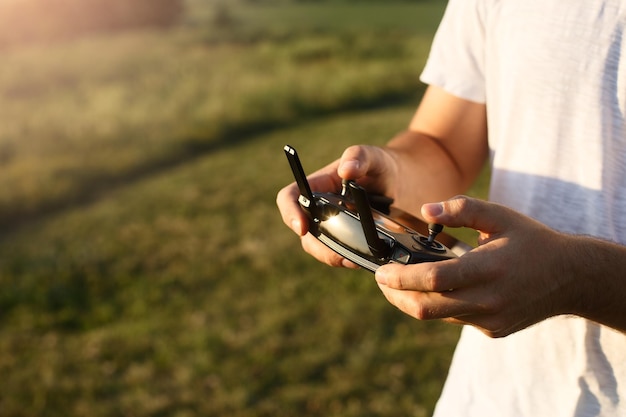The photograph captures a close-up of a person, likely male, holding a black controller in both hands. The controller features dual antennas and two joysticks, which the person is manipulating with their thumbs. The individual, who has light tan skin and is wearing a bone-white, short-sleeved t-shirt, appears to be standing in a sunlit outdoor setting with green grass visible in the blurred background. This suggests he might be operating a drone in a park or his yard. The focus is sharply on him and the device, emphasizing his engagement with the controller amid the sunny, grassy surroundings.